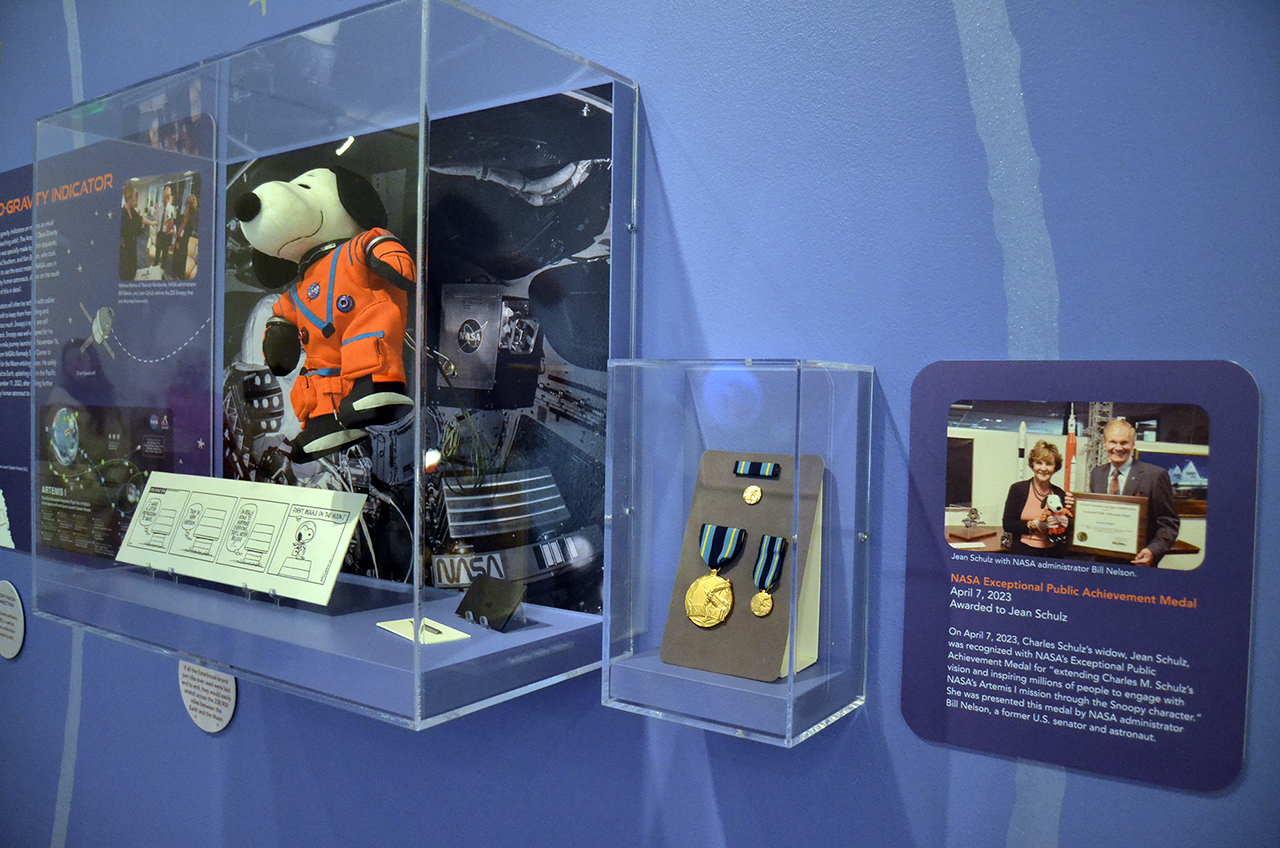The image depicts an indoor museum exhibit or display with various shades of light blue and medium blue on the walls, interspersed with white and silver-like lines. Central to the image is a large Lucite case mounted on the wall, containing a Snoopy doll clad in an orange astronaut suit complete with matching gloves. Behind Snoopy, the background appears to simulate space, accentuated by NASA insignias. Directly in front of the Snoopy doll is a black-and-white strip from the "Peanuts" comic, although the details are not clearly legible.

To the right of this setup, a smaller Lucite case houses three gold medals, each attached to ribbons with dark blue and light blue stripes. Adjacent to these, a navy-blue placard displays the images of a man and a woman - the man holding an award, and the woman clutching the Snoopy doll. The plaque is accompanied by explanatory white text, though the specifics are unreadable in the image. Further left, additional placards are visible, featuring more information in white and orange text. The meticulous arrangement and specific artifacts indicate that this display is part of an astronaut or space-themed exhibit, celebrating achievements related to space exploration.